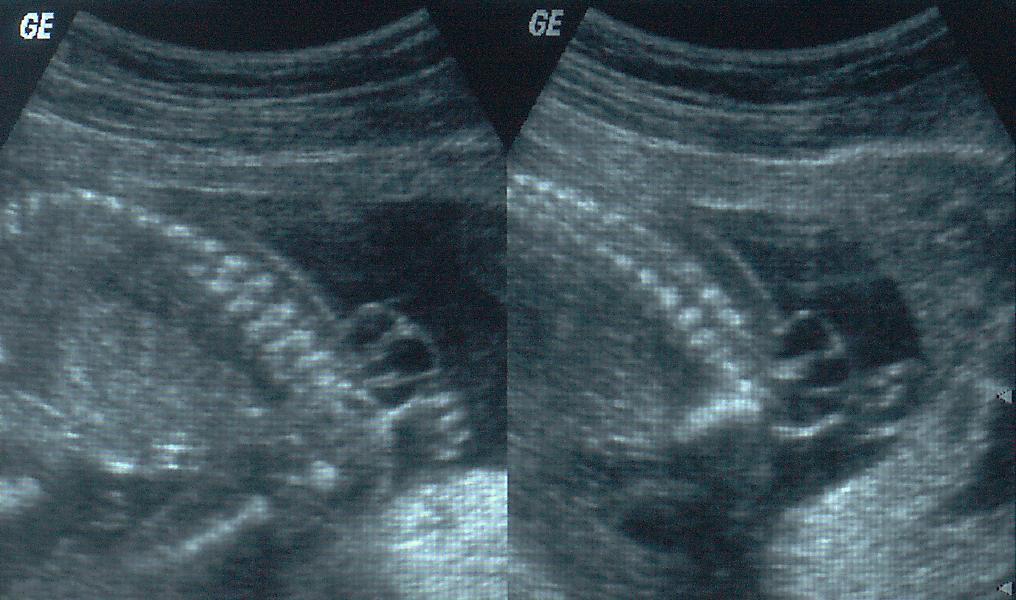This image displays two side-by-side black and white sonogram pictures created by General Electric, marked by the letters "GE" in the top corners of each section. The images, with their grainy, ultrasound texture, seem to depict a baby in early development stages. The main focal points in both sonograms are the baby's spine, which starts in the center and curves upward to the left, resembling a column of white dots akin to a spinal cord. Additionally, the images hint at the presence of hands and possibly other limbs, although distinguishing specific anatomical details remains challenging due to the sonogram's inherent lack of clarity. The background is predominantly black, enhancing the contrast and making the white and gray regions of the images more prominent. Overall, the sonograms provide a detailed look inside, revealing the curled-up form of a developing baby amidst various shades of gray.